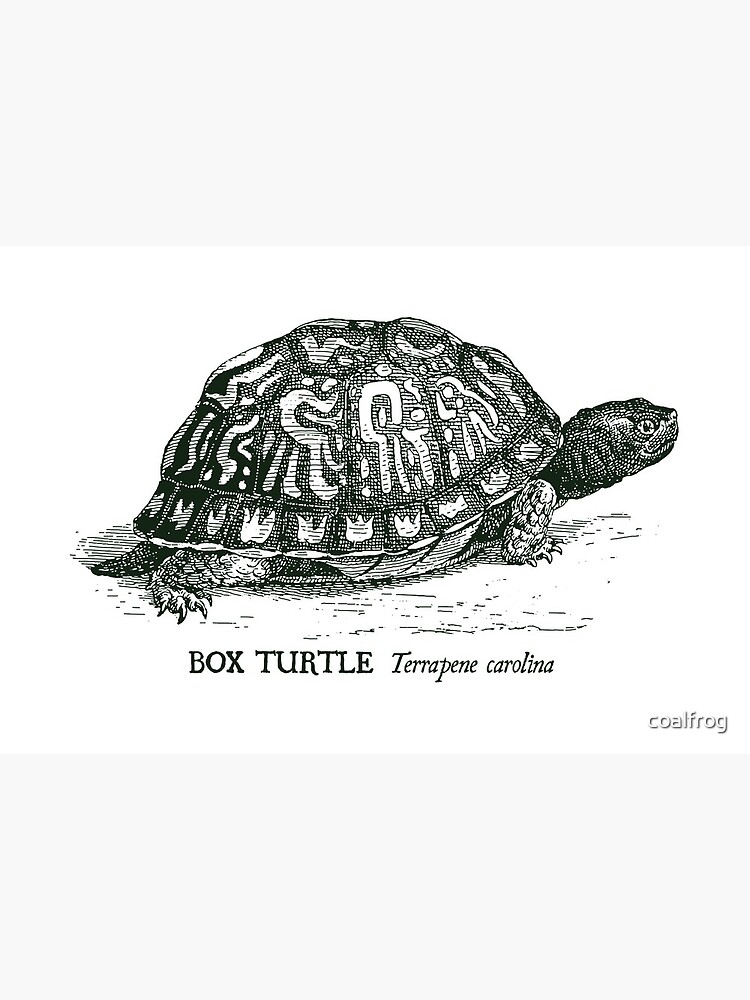This detailed black and white pencil drawing intricately depicts a box turtle, with the caption "Box Turtle" and the scientific name "Terrapene carolina" prominently displayed. The turtle, facing right with its head peeking out and appearing in motion, showcases beautifully abstract designs on its shell, including hieroglyphic-like patterns and dot designs that resemble small flames near the lower shell—almost crown-like. The meticulous texture of the turtle's scale-covered head and visible feet emphasize its forward movement. The image, which appears to have an all-white background reminiscent of a book cover or photo, bears a watermark in the lower right corner reading "Coal Frog."